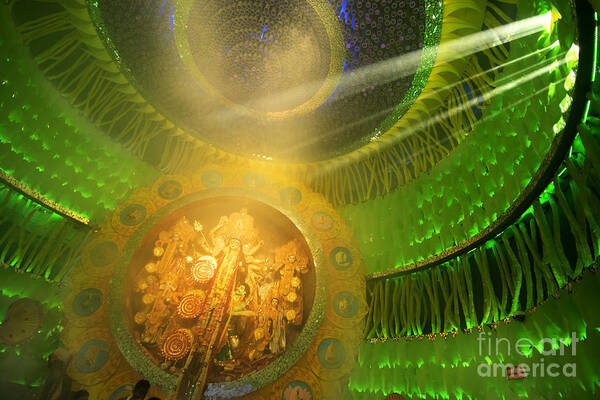This is a richly detailed color photograph of an ornate Indian temple interior. At its center stands a prominent gold statue of a Hindu goddess adorned with intricate, large headwear and multiple limbs, possibly six or eight. The goddess is elaborately designed and is the main focal point of the image. Surrounding her, the temple's spherical interior is illuminated with lime neon green lights and decorated with elaborate jewels at the roof's peak. Small, white, pillow-like ornamentations hang from the temple structure, adding to the ornate ambiance. The ceiling displays a circular pattern with a brown center, bordered by yellow and bluish-black rings. In the lower-left corner of the image, a golden medallion with green accents can be seen, reminiscent of a religious relic. The overall scene is characterized by a vibrant mix of greens, yellows, blacks, and oranges, creating a mesmerizing and intricate visual experience. In the lower right-hand corner, the words "fine art, America" subtly suggest the artistic nature of the representation.